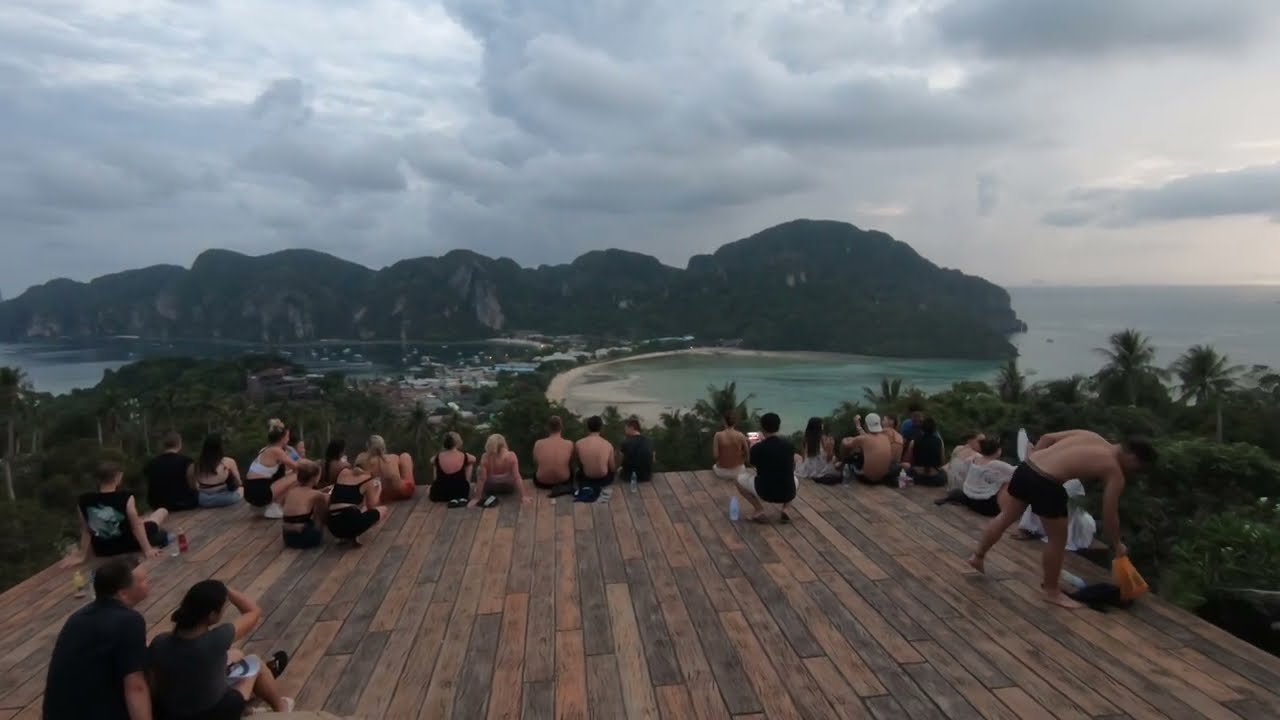The image portrays an overlook patio made of various shades of light and dark brown wooden planks, arranged in a square shape. It sits elevated above an island's bay, providing a vantage point from which several people, dressed in swimsuits and casual summer attire, sit with their backs to the camera. They are looking out over a stunning vista that includes a docking area on a narrow strip of land, where several white boats are docked near small, flat-roofed, rectangular buildings. Behind this, low-lying mountains dotted with lush green vegetation and patches of white stone frame the scene. The cloudy gray sky above hints at an overcast day without any visible sunlight, adding a soft, diffused light to the landscape. Palm trees and other tropical vegetation add to the exotic feel of the locale. The image captures a tranquil moment as the viewers on the patio take in the expansive view of the turquoise waters and the mountainous shoreline stretching into the distance, enveloped in a serene, cloudy atmosphere.